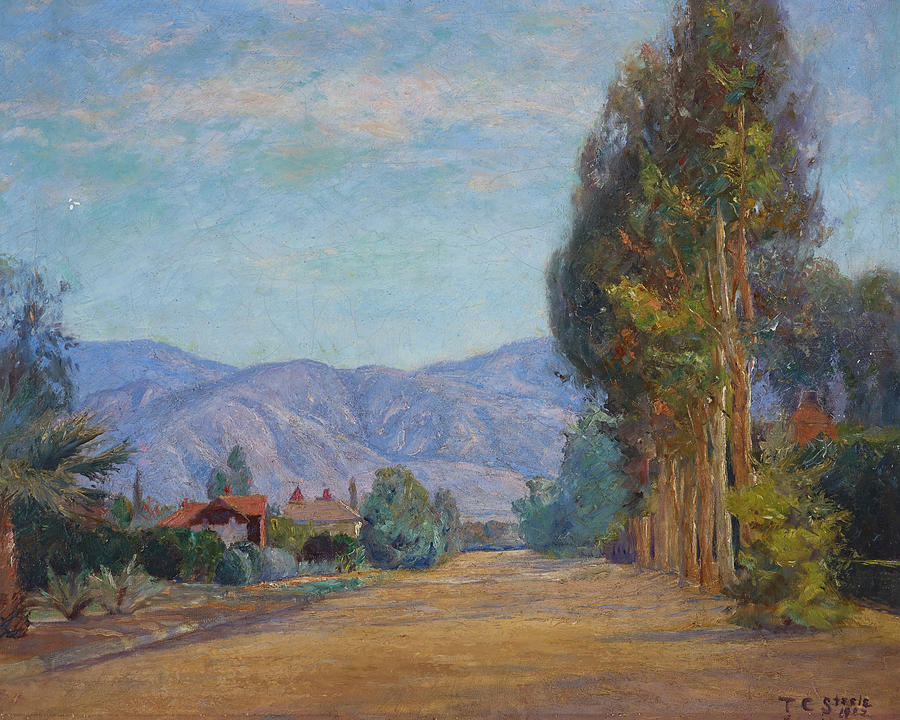The painting depicts an old-timey, tranquil rural scene with a central dirt road leading towards a mountainous backdrop. On the right, a row of tall, vibrant fall trees and shorter bushes border the path, extending into the distance. To the left, two small houses with visible chimneys nestle among lower trees and shrubs. The rugged mountain range in the background is detailed with trees and darker foliage that accentuate its cracks and crevices. The sky above is a clear blue adorned with scattered clouds in shades of peach, tan, gray, and darker blue hues, adding depth and atmosphere to the serene landscape. The terrain hints at an arid, possibly South American setting, with its brown, desert-like ground and sparse, varied vegetation.